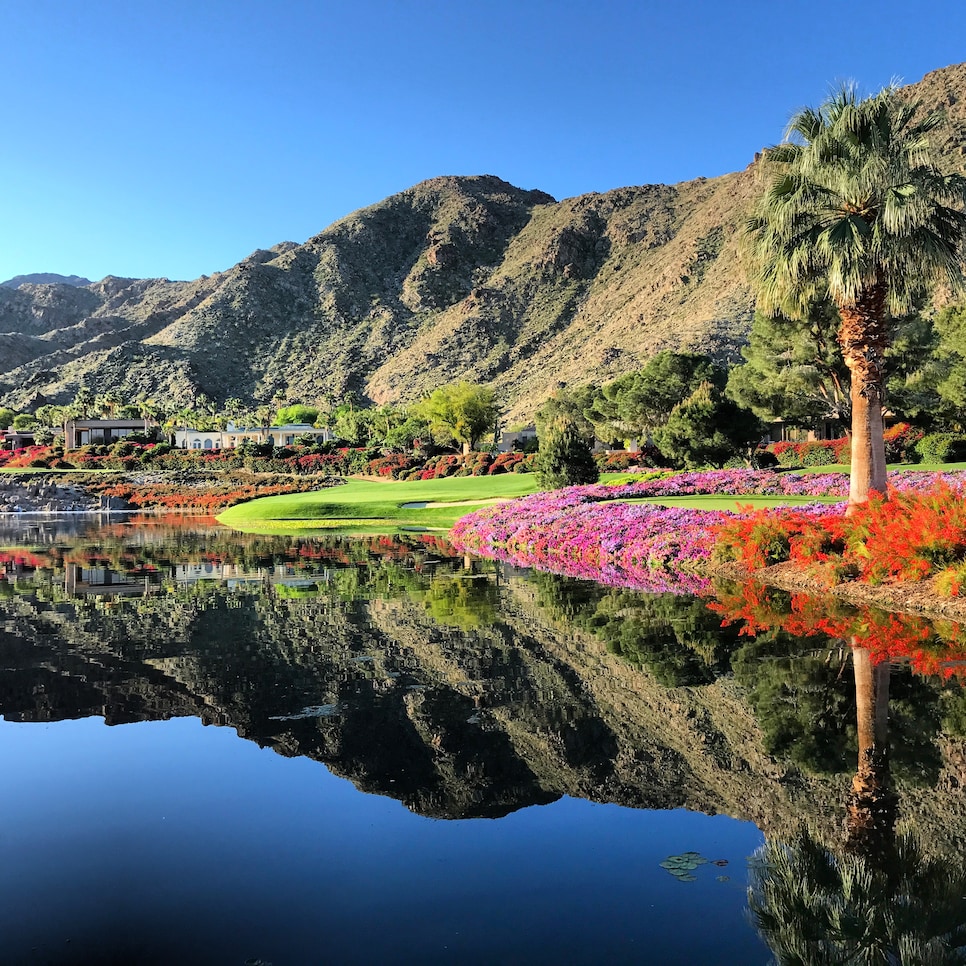A vibrant mountainside property is depicted in this picture. The background features bumpy, rolling mountains in varying shades of green against a bright, cloudless blue sky. At the base of these mountains lies a dense cluster of trees, leading to two notable houses near the water. One is a large, brown house, and the other is a lighter-colored structure surrounded by lush foliage and red flowers. The foreground showcases bright green grass, reminiscent of a well-manicured golf course, adorned with a circular arrangement of vivid pink and red flowers, with a towering palm tree at the center. Additionally, a large, tranquil body of water graces the scene, reflecting the mountains, flowers, and palm tree, adding to the idyllic ambiance.